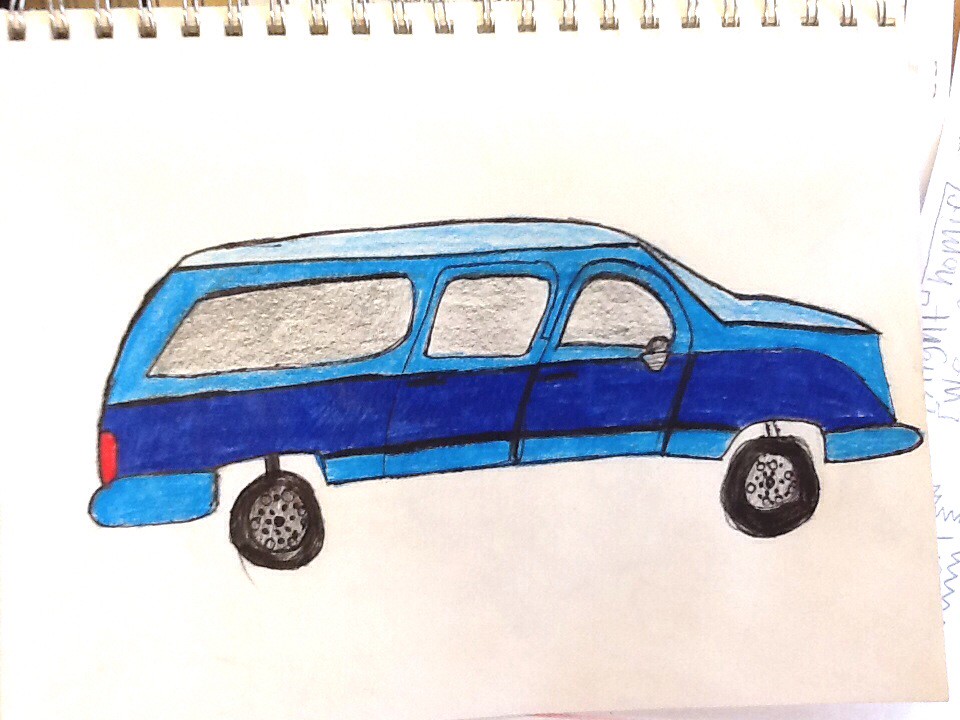This is a charming and detailed child's drawing of a vintage station wagon or small van. The vehicle is depicted with three visible windows and a two-tone color scheme featuring a very light blue body accented by a striking blue streak that runs from the front to the back. Although the car is void of any occupants, it stands out with its meticulous detailing. The two visible black tires are slightly out of proportion, with circular bolts adorning the rims. The rear of the vehicle is highlighted with a prominent red taillight, enhancing the overall appeal of this talented young artist's creation.